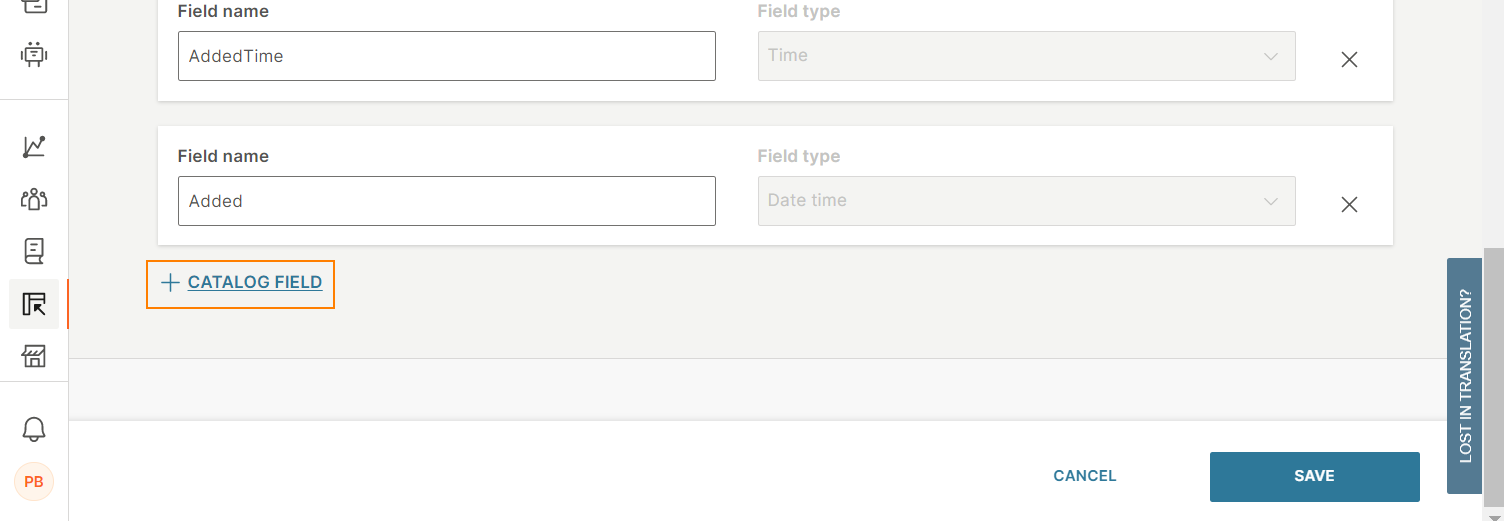In this image, categories are displayed on the left-hand side, arranged into three distinct sections: two categories at the top, five in the middle, and two at the bottom. Each category is represented by a small emblem, with the bottom-most emblem marked "PD" in red. To the right of these categories, there are four fields of information organized vertically. 

The top field contains the label "Name" followed by "Added Time," with the field type "Time" listed to the right. Below this is another field with the label "Name" followed by "Added," and the field type "Date Time" to the right. Directly beneath these is a rectangular section outlined in orange, featuring the label "Catalog Field" displayed in blue text. The background of this entire area is shaded in gray.

At the bottom of the image, two buttons are present: a "Cancel" button in blue on the left, and a "Save" button in a dark blue rectangle on the right. Additionally, a scroll bar on the far right side of the screen is visible, scrolled all the way to the bottom. This comprehensive layout completes the visual from top to bottom.